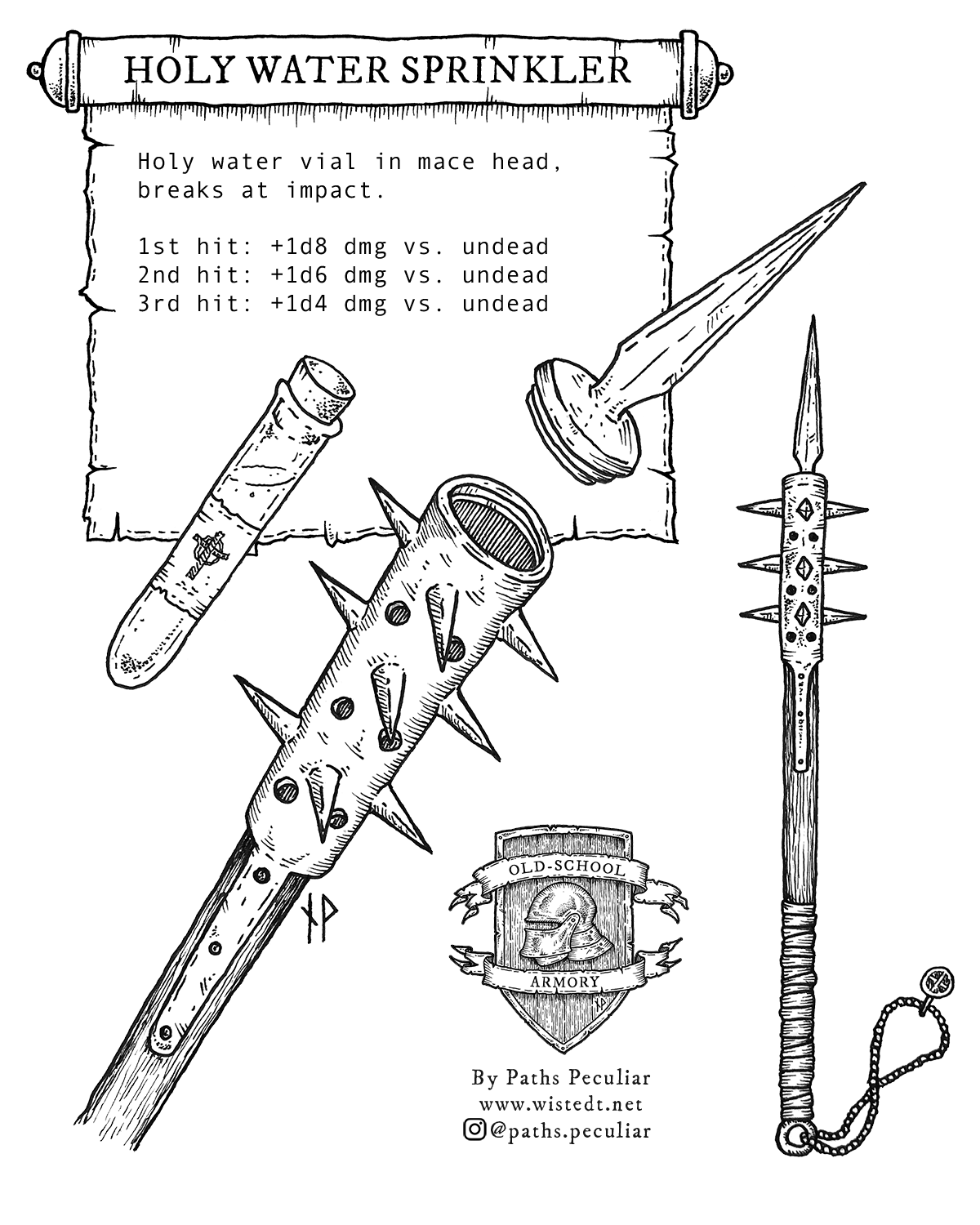This detailed ink illustration, set against a completely white background, showcases a unique medieval weapon labeled as the "holy water sprinkler." The title is elegantly drawn on a scroll halfway down the image, which includes intricate text describing its effects: "holy water vial in mace head breaks at impact. First hit: +1d8 dmg versus undead. Second hit: +1d6 dmg versus undead. Third hit: +1d4 dmg versus undead." 

The illustration features a complex design for the weapon. It incorporates a segmented mace that unscrews to reveal a hollow chamber within the spiked head, designed to house a corked vial of holy water featuring a small cross. Detailed instructions indicate that the mace's head can be opened, revealing a pointed spear tip where the vial is inserted. When closed, the mace displays a formidable array of spikes and a cross-adorned chain, with a leather-wrapped handle for secure grip.

Adjacent to the weapon are additional elements: a plaque symbolizing the "old school armory" by Paths Peculiar, along with a web address, www.wistedt.net, and an Instagram handle, @paths.peculiar. The artistry and detail hint at a historical or fantasy context, possibly for use in games like Dungeons & Dragons, showcasing a blend of practicality and imaginative design.